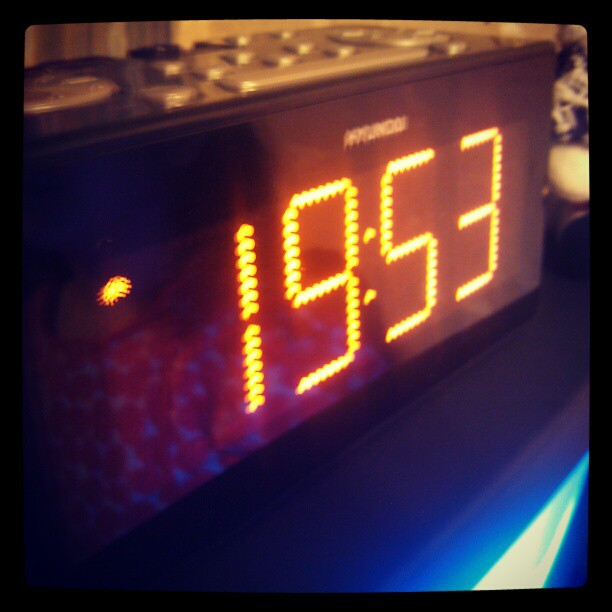The photograph features a sleek, black, rectangular alarm clock positioned at a slight diagonal angle. Dominating the front of the clock, the digital display shows the time as 19:53. Adjacent to the time display, a small red indicator light is illuminated in the top left corner. The clock's uniform black finish enshrouds a series of unlabeled, variably shaped buttons adorning the top panel. Above the time display, a white logo is faintly visible but appears too blurry to identify. The alarm clock rests on a blue surface, possibly a table, with some indiscernible fabric faintly visible in the background, adding a touch of texture to the setting.